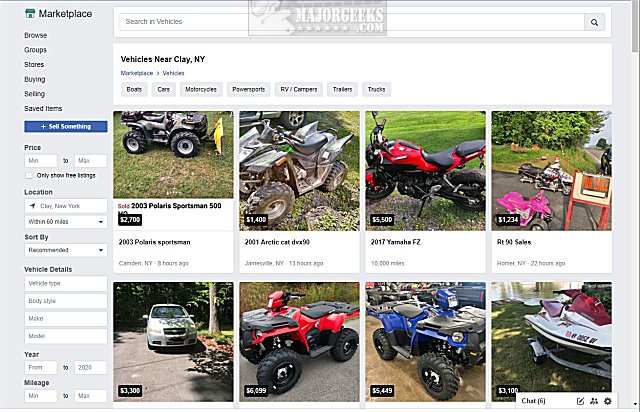**Detailed Caption:**

This screenshot captures an online marketplace interface focused on motorized vehicles. The central section displays a variety of listings including ATVs, a motorcycle, a dirt bike, and a jet ski. Notably visible among these are a red ATV and a blue ATV. 

On the right side, a detailed search panel allows users to filter vehicles based on various criteria: price range (minimum to maximum), location (within a specified mile radius), and sorting options (e.g., recommended listings). Additionally, users can input specific vehicle details such as the year and mileage to refine their search. 

At the top of the interface, a navigation bar provides quick access to categories including vehicles near Clay, New York, cars, motorcycles, power sports, RV campers, trailers, and trucks.